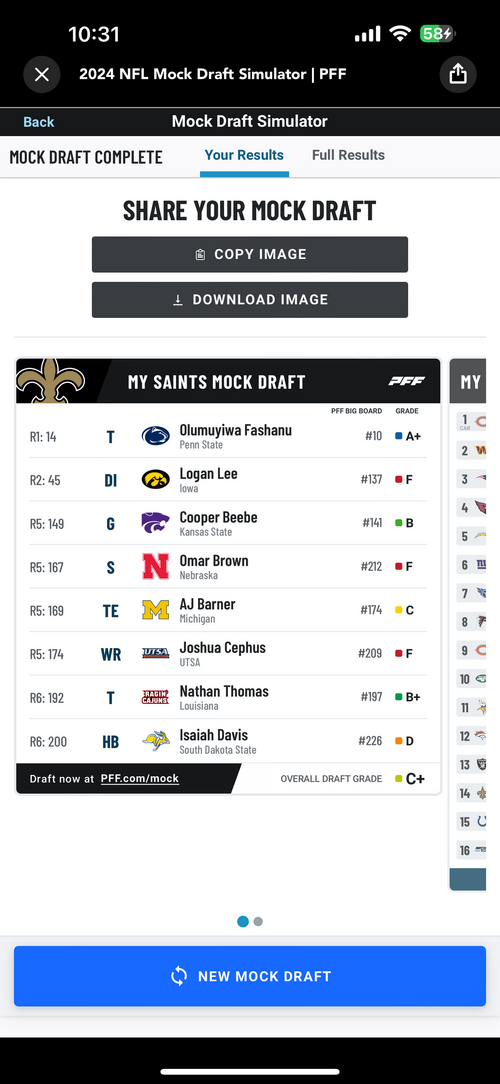This image is a mobile screenshot of a completed 2024 NFL mock draft from the PFF mock draft simulator. The screenshot, taken at 10:31 AM with the battery at 58%, captures a detailed summary of the user's picks for the Saints. The top of the image features a black bar with the time and battery status, followed by the title "2024 NFL Mock Draft Simulator PFF". Below this, the interface shows a navigation bar with "Mock Draft Complete" on the left and the underlined "Your Results" in blue, and "Full Results" to the right. In large, bold, black capital letters is a prompt to "SHARE YOUR MOCK DRAFT". 

Two grey buttons labeled "Copy Image" and "Download Image" are positioned just below the prompt. The main content features the heading "My Saints Mock Draft" accompanied by the Saints logo. The selected players and their details are listed as follows:

1. **R1 14T**: Olumayuwa Foshanu, Penn State - Grade: A+
2. **R2 45TI**: Logan Lee, Iowa - Grade: F
3. **R5 149G**: Cooper Beebe, Kansas State - Grade: B
4. **R5 167S**: Omer Brown, Nebraska - Grade: F
5. **R5 169TE**: AJ Barner, Michigan - Grade: C
6. **R5 174WR**: Joshua Cephas, UTSA - Grade: F
7. **R6 192T**: Nathan Thomas, Louisiana - Grade: B+
8. **R6 200HB**: Isaiah Davis, South Dakota State - Grade: D

The overall draft grade given is a C+.